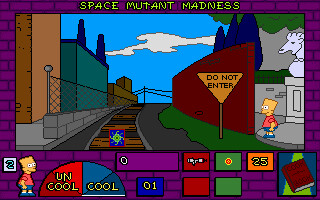This is a detailed screenshot from an older Simpsons video game, likely from the 1990s. At the top of the screen, "Space Mutant Madness" is prominently displayed in fluorescent green text. The main section of the image features Bart Simpson about to enter a "Do Not Enter" area. The left side of the image shows a train track, while the right side focuses on Bart. Bart is dressed in an orange T-shirt, blue shorts, blue shoes, and white socks. Behind Bart is a building that resembles a library, featuring a stone bust of what looks like a lion in shades of light and dark gray.

At the bottom, there is an indicator for Bart's status, divided into "Uncool" and "Cool," with "Uncool" on a red background and "Cool" on a blue background, formatted in a semi-circle split down the middle. On the right side of the screen, there is an inventory display showing Bart with a squirt gun, some coins, and what appears to be a diary or ledger.